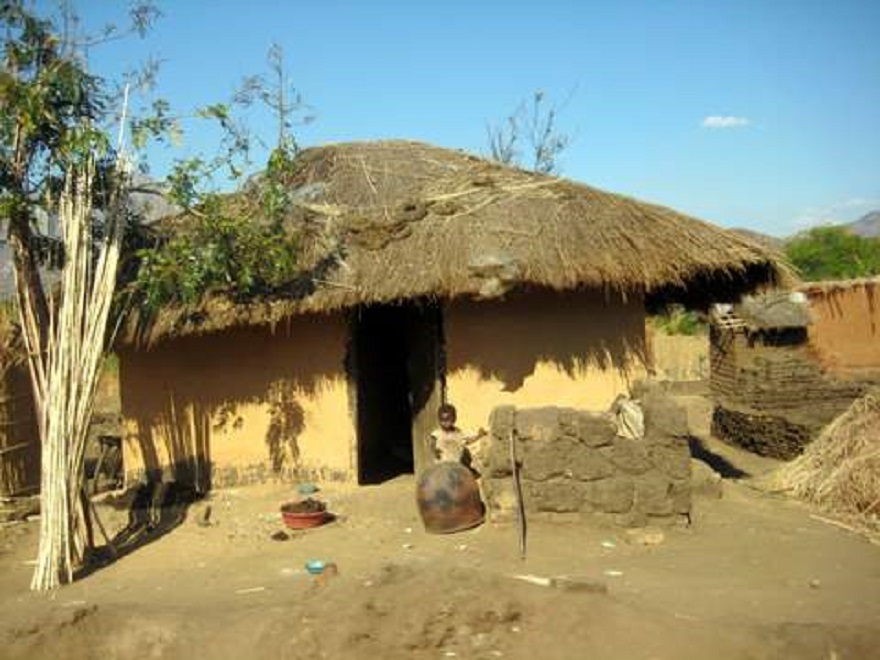The image showcases a small, yellow clay or brick hut with a thatched roof, prominently centered in the photograph. The roof is made of straw, and the ground in front of the hut is bare dirt. The slightly ajar front door reveals only darkness within. Standing in front of the door is a small black child with dark hair, wearing a light-colored frock. Next to the child is an overturned metal pot and a modest stone wall.

To the left of the hut is either a tree or a bundle of sticks that extends above the roof, featuring some brown, tan, and white hues with a bit of green foliage at the top. In the background, the blue sky with one small white cloud can be seen on the right, along with some green landscapes and possibly distant mountains. On the right side of the hut, there is a trench, another small building or enclosure, and a pile of hay or thatching. Scattered about the ground in front of the hut are a tiny blue bowl and a terracotta pot with some soil.